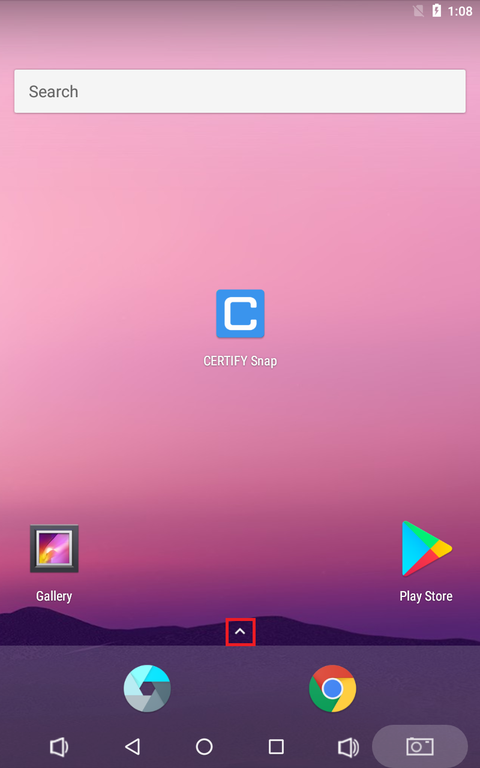This image depicts the home screen of a Google mobile device. The device's screen is predominantly rectangular, showcasing a vibrant background image with a pink and purple gradient reminiscent of a serene sunset. At the top right corner, a battery icon indicates the current battery level, and the time displayed is 1:08.

Centered towards the upper portion of the screen is a white search box with the prompt "Search" written in grey text. Dominantly positioned in the middle of the screen is a blue square icon featuring a white letter 'C' within it, labeled "Certify Snap."

Directly below this icon, near the lower section of the screen, is a prominent upward-facing caret highlighted by a red square, likely intended to draw the user's attention to it for potential interaction.

To the left of the caret is a square icon with the label "Gallery" beneath it, suggesting a shortcut to the device's photo gallery. Adjacent to the right is the Play Store icon with the text "Play Store" below it for quick access to Google's app marketplace.

The footer bar includes two circular icons: one resembling a camera and the other a chrome icon, possibly for web browsing. Below the footer bar, there is a series of smaller icons representing various functions, including volume controls, media playback options, and a camera, providing quick access to these essential utilities.